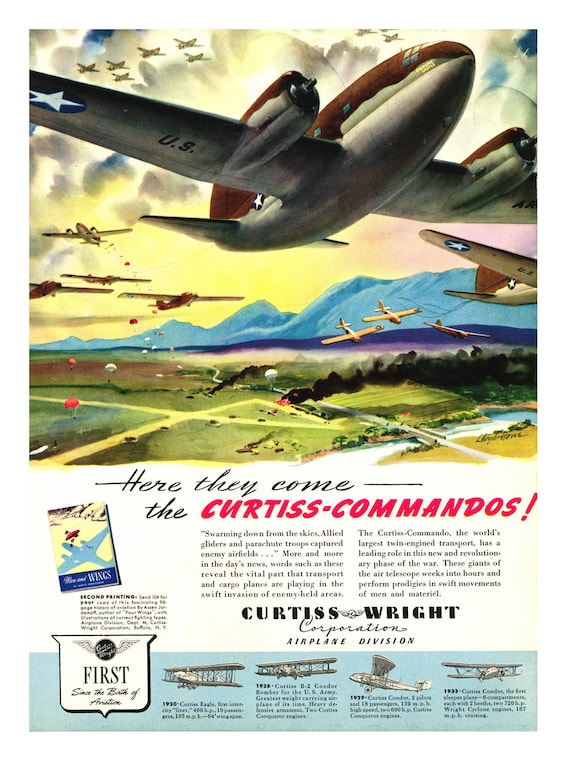This colored print advertisement for the Curtis-Wright Corporation Airplane Division, likely from the World War II era, showcases the pivotal role of their aircraft in the Allied efforts. Dominating the top half of the ad is a vivid illustration, possibly rendered in watercolor, depicting a variety of U.S. military planes adorned with the distinctive U.S. insignia—a white star encircled in blue. These aircraft are depicted soaring through a tropical landscape underlain by blue mountains, with paratroopers descending to the ground amidst smoke and fire, suggesting ongoing battles and crashed planes below.

The scene is dynamic, capturing the moment Allied gliders and parachute troops are taking control of enemy airfields, a testament to the crucial impact of transport and cargo planes like the Curtis Commando. The ad's text emphasizes the importance of these airplanes in accelerating the invasion of enemy-held territories by stating, “Here they come, the Curtis Commandos," and elaborating on the transformative speed and efficiency the world's largest twin-engine transport brings to military operations. A medallion proclaiming "First, since the birth of aviation," and historical references to early airplanes from the 1920s also feature at the bottom, reinforcing the brand’s longstanding aviation heritage. This advertisement most likely appeared in a magazine, underscoring Curtis-Wright's contribution to the war effort.